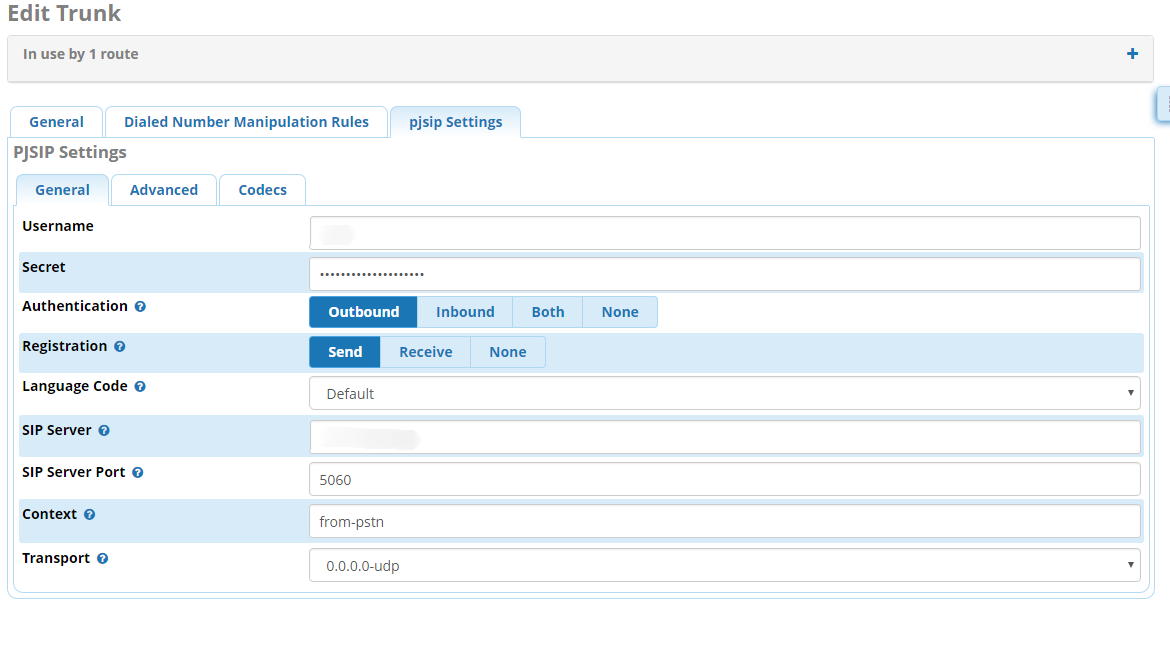The image displays a detailed interface of a telecommunication software configuration screen. 

In the top-left corner, there's a gray screen labeled "Edit Trunk." Directly beneath it, there is a gray bar containing the text "In use by one route" written in gray lettering, spanning across the bar with a plus mark.

Directly below this bar, there is a section titled "Files." At the very top are several tabs labeled: General, Dialed Number Manipulation Rules, and PGSIP Settings. The currently opened tab is PGSIP Settings.

Inside the PGSIP Settings tab, this title appears in gray, all uppercase letters at the very top. Beneath this heading, additional sub-tabs are visible: General, Advanced, and Codecs. The General sub-tab is active, detailing several fields:

- **Username** (not filled in)
- **Secret** (contains typed information)
- **Authentication** (followed by outbound settings)
- **Registration** (options to send registration)
- **Language Code** (set to default)

The section also includes information about the SIP server:
- **SIP Server** (grayed out)
- **SIP Server Port** (set to 5060)
- **Context** (set to from PSTN)
- **Transport** (showing a series of numbers in USDP)

All sections, except for 'Secret', have an accompanying question mark icon, indicating that users can click on it for further information to properly complete the fields.